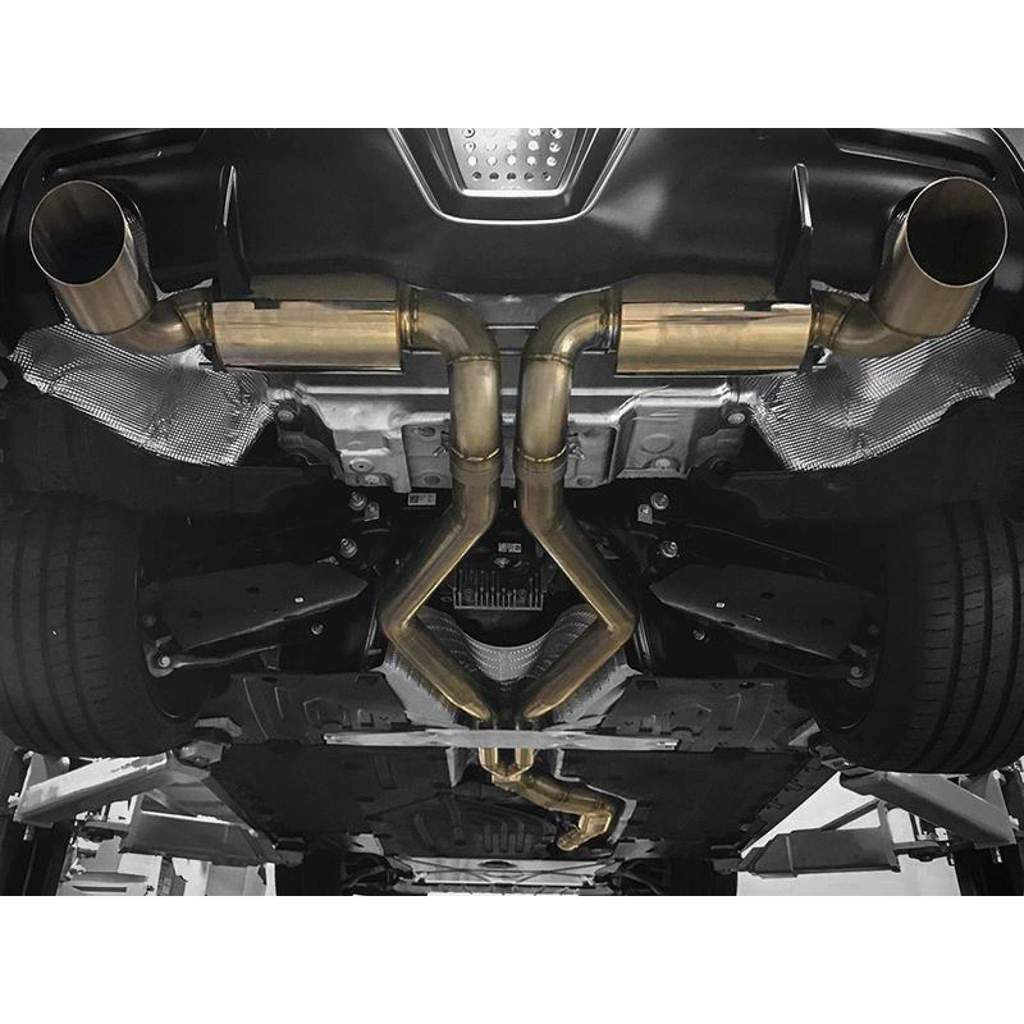This image displays a meticulously clean underside of a vehicle, raised on a mechanic's lift. Dominating the view is a newly installed dual exhaust system. The pipes, slightly gold-tinted, extend from the back of the vehicle, where they are connected to drum-shaped mufflers. These pipes run parallel to each other along the middle of the car, creating a diamond-like pattern before they sharply turn outward and then merge into a single larger pipe towards the front. The underside appears spotless, with no speck of dirt visible, highlighting either the newness of the car or a thorough cleaning. Visible components around the exhaust system include silver accents, while the rest of the undercarriage is largely black. The car's rear tires, which show minimal wear, are thick and visible toward the bottom and edges of the image. The entire underside and parts of the lift, in light gray, dominate the image with dark grays, blacks, silver, and goldish hues.